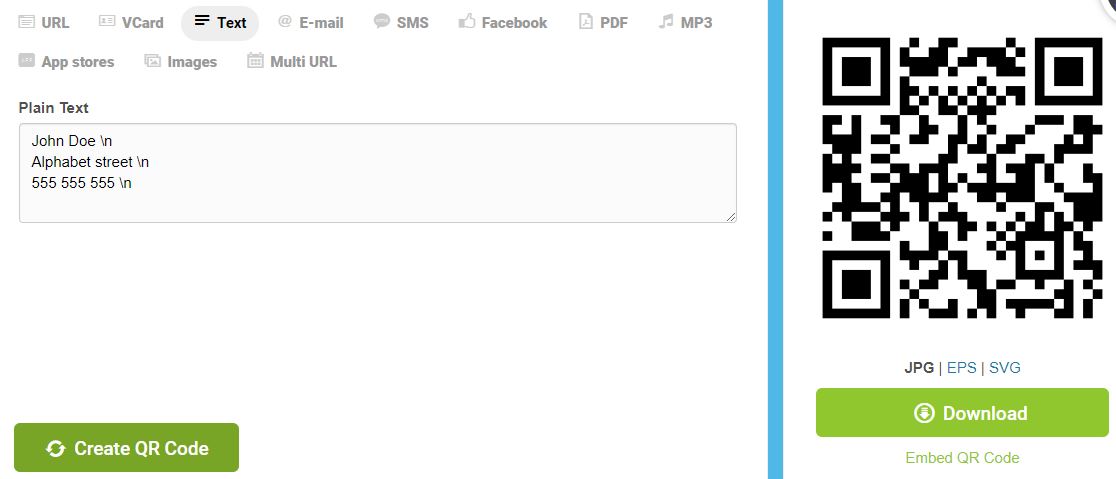The image is a screenshot of a two-pane user interface. The left pane functions as a menu bar and comprises two rows of options, each accompanied by an icon. The first row lists "URL," "V Card," "Text," "Email," "SMS," "Facebook," "PDF," and "MP3," while the second row includes "App Store," "Images," and "Multi-URL." The "Text" option, situated third from the left in the first row, is highlighted, indicating it is selected.

Directly below the menu bar, there is a plain text input box containing the text:
```
John Doe
Alphabet Street
555-555-5555
```
This text is presumably the data to be encoded into the QR code. At the bottom left of the pane, a green button labeled "Create QR Code" is prominently displayed.

A vertical blue divider separates the left pane from the right. To the right of this divider is the generated QR code. Directly beneath the QR code, there is a row listing the file formats "GPG," "EPS," and "SVG" for download options. Below this row, a green "Download" button is present, followed by the text "Embed QR Code" in green.

The overall layout is designed to allow users to input data, generate a QR code, and provide various download and embedding options for the generated code.